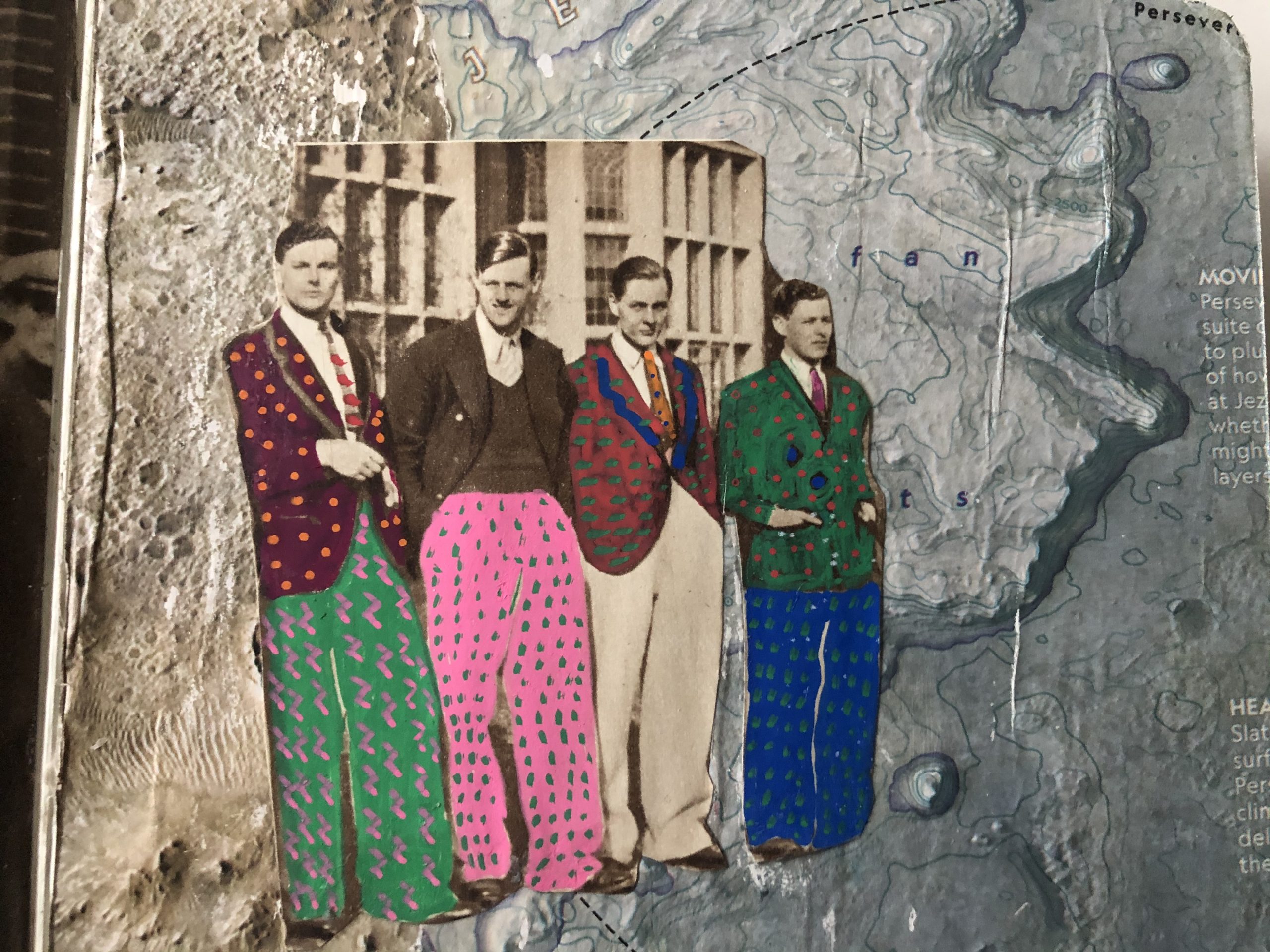This image appears to be a meticulously crafted collage featuring a vintage, early 1900s photograph of four men in suits, positioned against a background of a black-and-white topographical map. The map, which includes craggy, moon-like terrain in a sepia tone on the left side, has partially visible text, including the word "Persevere" in the upper right corner. The photograph of the four men in front of a building is prominently altered with vividly hand-painted, new-wave attire: 

- The man on the far left sports a purple jacket with orange spots and green pants adorned with pink zigzags. 
- The second man retains his original suit jacket but now wears pink pants featuring blue dots. 
- The third man wears a brown or red jacket with green dots and blue trim, a tie with orange accents, and his original sepia-toned pants. 
- The fourth man is dressed in a green jacket with orange dots and blue buttons, a red or purple tie, and blue pants with green dots.

Their colorful, almost whimsical attire contrasts sharply with the antiquated and sober feel of the original photograph and the black-and-white map background, creating a captivating juxtaposition.